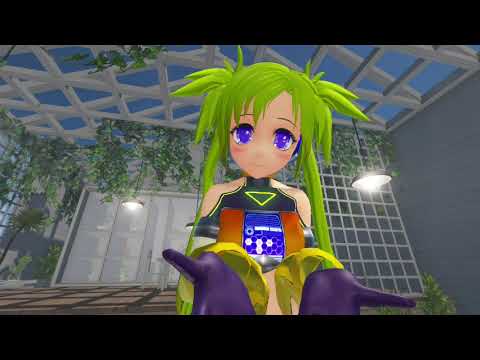The image depicts a vividly rendered scene from a digital game, featuring a young, three-dimensional female character with a striking appearance. The character has short, bright green spiky hair that extends longer in the back, large, bright purple eyes, and rosy cheeks. She wears a distinctive outfit in black, red, and blue, adorned with an emblem on her chest resembling cellular or brain designs, hinting at a superhero or scientific theme. She also sports purple gloves and is holding her hands out in front of her as if offering something.

The backdrop is a bustling greenhouse with a roof supported by white beams, filled with plants and vines that cascade down the walls. To the right is a gray gate, while to the left, there is an entrance. The scene is bathed in daylight, visible through the roof, accentuating the bright and vibrant atmosphere. The overall image is clear, capturing intricate details that enhance the animated character's lively and engaging demeanor. A ceiling light on the right side further illuminates the setting, adding to the well-lit environment.